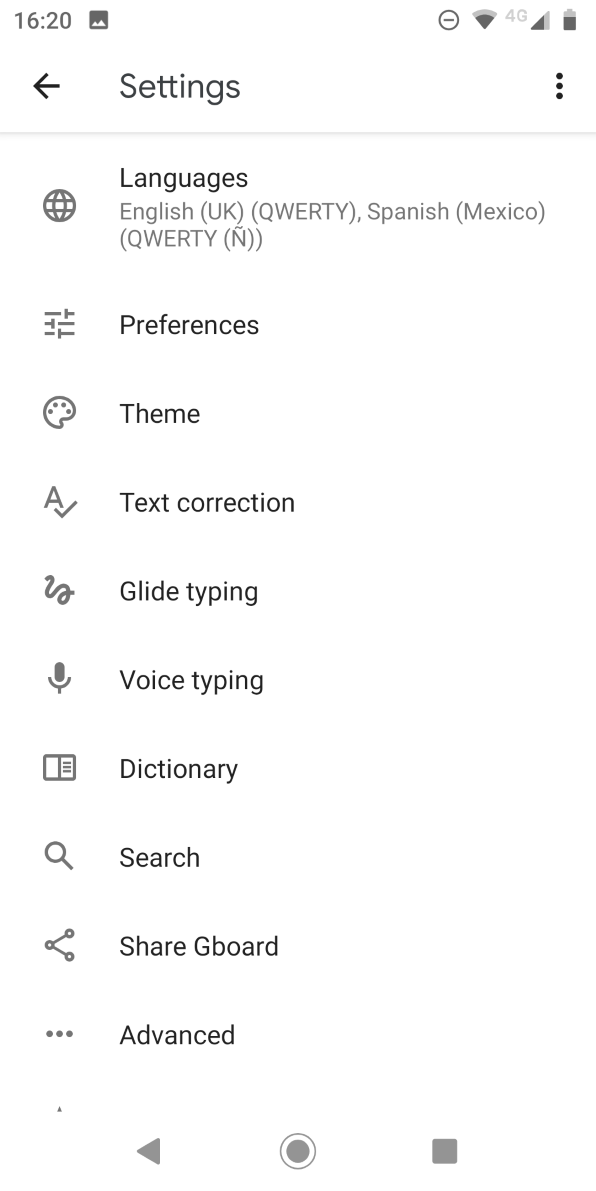The image showcases the "Settings" section of a smartphone screen, captured at 16:20 hours. At the top of the screen, several icons are visible: on the left, a back arrow, and on the right, indicators for battery life, 4G signal, and a trio of vertically aligned dots, which suggest a menu option.

Below this top bar, the "Settings" menu is divided into several sections. The first section features a globe icon next to the word "Languages," listing options such as "English (UK) - QWERTY" and "Spanish (Mexico) - QWERTY". Following this, there are various other settings denoted by distinct icons and labels:

- A series of horizontal lines with hashes labeled "Preferences."
- An artist's palette icon next to the word "Theme."
- A checkmark beside an uppercase "A" indicating "Text correction."
- A squiggly line representing "Glide typing."
- A microphone icon denoting "Voice typing."
- A book with text, labeled "Dictionary."
- A magnifying glass symbolizing "Search."
- A sideways "V" indicating the option to "Share Gboard."
- A three-dot menu titled "Advanced."

At the very bottom of the screen, the navigation bar contains the standard Android interface icons: a triangle for "Back," a circle for "Home," and a square for "Overview."